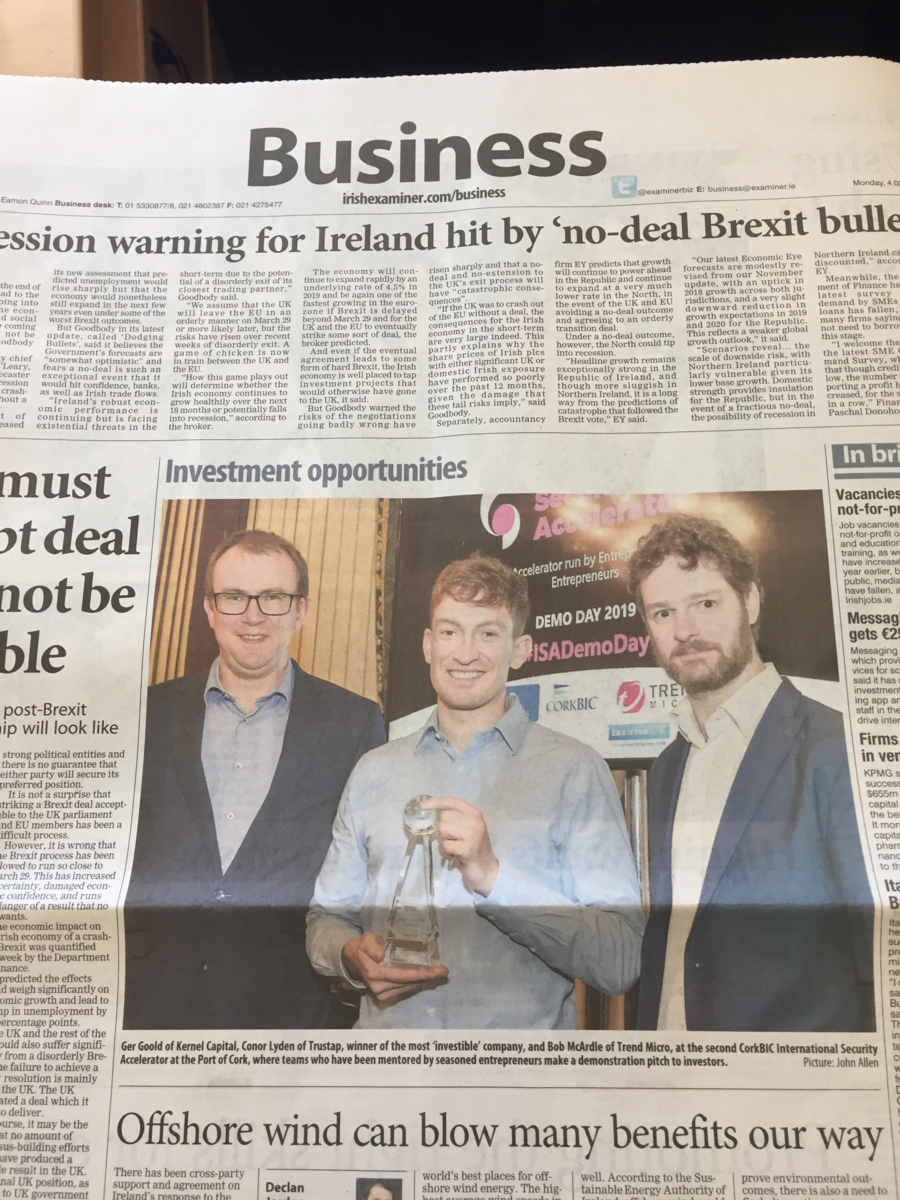Front page of the Business section of the Irish Examiner

The Business section of the Irish Examiner, found at irishexaminer.com/business, features a predominantly black-and-white layout with a large, central color photograph. The vibrant image depicts a young man receiving a glass trophy from two older gentlemen, celebrating an award ceremony. Above the photo, the headline reads "Investment Opportunities." At the very top of the page, an article titled "Session Warning for Ireland Hit by No Deal Brexit" is prominently displayed. Another headline on the page reads "Offshore Wind Can Blow Many Benefits Our Way," indicating a focus on renewable energy. The placement and striking color photo make the page visually engaging amidst the text-heavy layout.